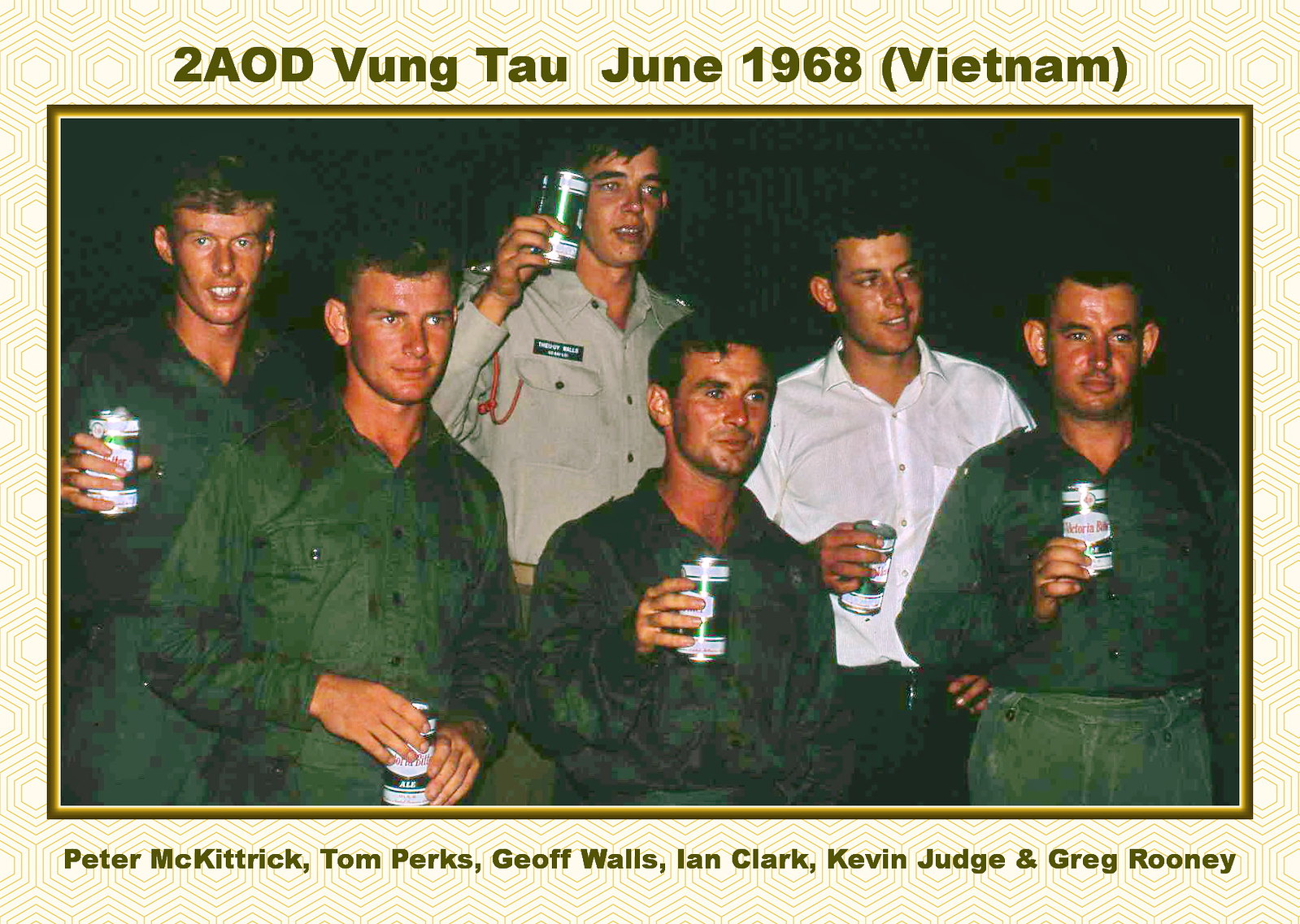In this rectangular photograph bordered by a geometric pattern in white and gold with a thin gold border around the image, six men are featured. The top of the photograph bears the inscription "A02AOD, Vung Tau, June 1968 (Vietnam)" in dark green letters. The bottom border lists their names: Peter McKittrick, Tom Perks, Geoff Walls, Ian Clark, Kevin Judge, and Greg Rooney. The men are positioned in two rows; four in the front are wearing green army uniforms, while in the back, one man is dressed in a light gray shirt, and the other in a white button-up shirt. All of them, appearing to be white men, are holding cans of what looks like beer, identifiable by their white and green cans. The background features a repeating hexagonal design and is black, suggesting the photo might have been taken at night.